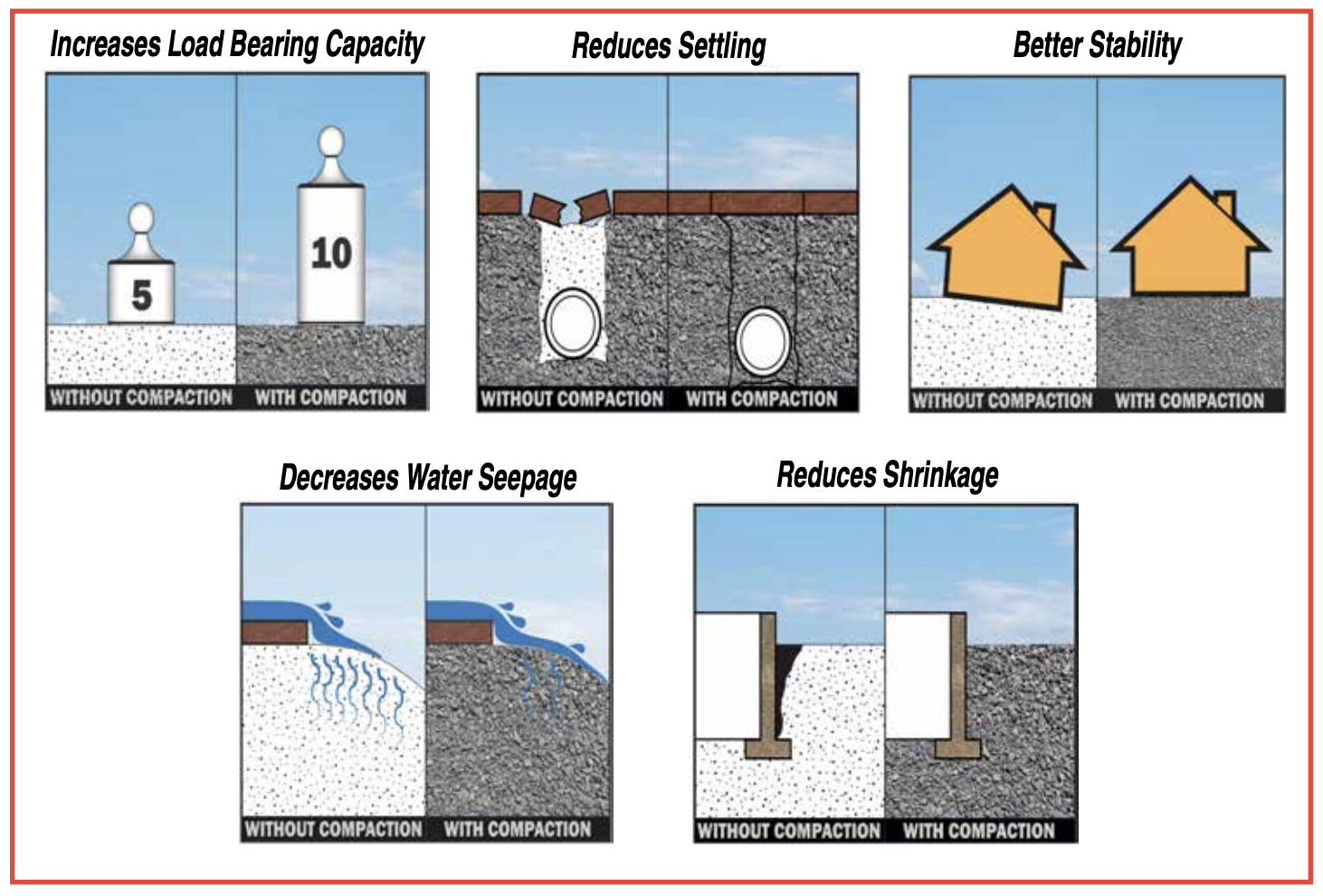The image appears to be a comparison chart, possibly from a booklet or PowerPoint slide, designed to highlight the benefits of soil compaction. It features five smaller images arranged in a grid on a white background with a thin red border. Each sub-image is captioned to illustrate specific advantages of soil compaction, with each benefit contrasted by showing conditions "without compaction" and "with compaction."

1. **Increases Load-Bearing Capacity**: The top left image compares two weights on the ground. The "without compaction" side shows a 5-pound weight, while the "with compaction" side shows a 10-pound weight, indicating that compaction increases the ground’s load-bearing capacity.

2. **Reduces Settling**: The top middle image depicts an underground white oval object with the ground surface above it. The "without compaction" side shows the ground cracked, whereas the "with compaction" side shows an intact surface, demonstrating reduced settling.

3. **Better Stability**: The top right image addresses structural stability, showcasing a house. The "without compaction" side illustrates the house slanting into the ground, while the "with compaction" side shows the house standing level and stable.

4. **Decreases Water Seepage**: The bottom left image contrasts water flow. The "without compaction" side shows water penetrating the ground, whereas the "with compaction" side shows water flowing over the surface, thus reducing water seepage.

5. **Reduces Shrinkage**: The bottom right image focuses on soil shrinkage. The "without compaction" side displays a noticeable black gap in the soil, while the "with compaction" side shows the soil intact and consistent, indicating reduced shrinkage.

Overall, the image clearly demonstrates through visual contrasts and descriptive captions how soil compaction can enhance load-bearing capacity, minimize settling, improve stability, decrease water seepage, and reduce soil shrinkage.